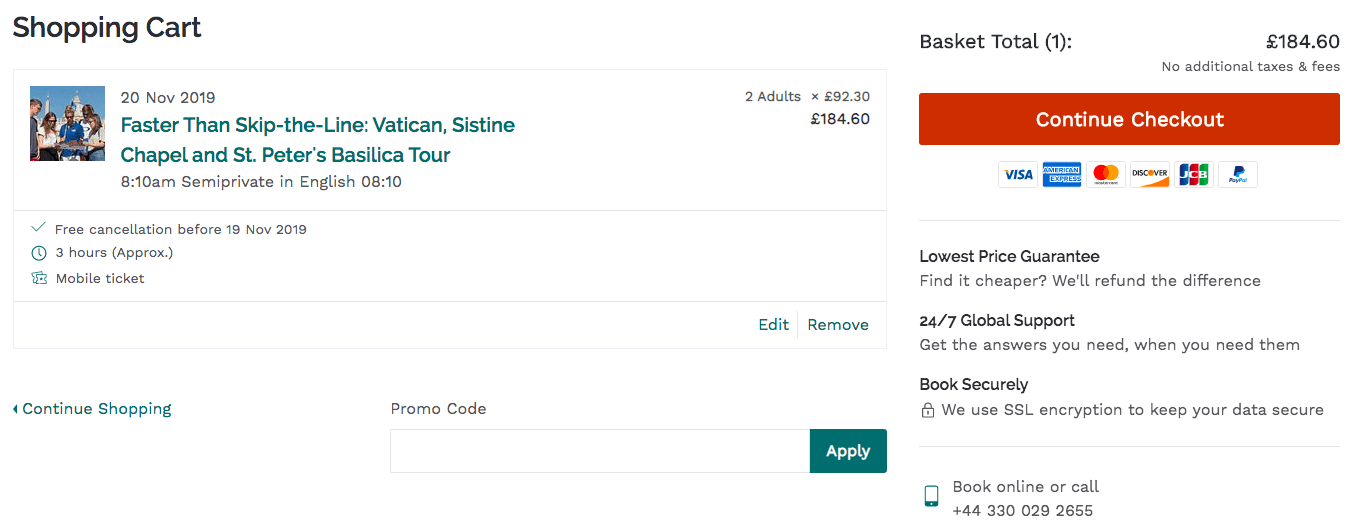This image depicts a website's shopping cart section with a clean, white background. In the upper left corner, the title "Shopping Cart" is displayed in black text. Below the title, the cart lists a tour booking titled "Faster than Skip-the-Line: Vatican, Sistine Chapel, and St. Peter's Basilica Tour" dated 20th November 2019 at 8 AM. Described as a "semi-private" English tour for two adults, the cost is £92.30 per person, totaling £184.60.

The booking details also mention a free cancellation policy before 19th November 2019, a total tour duration of approximately three hours, and that it is a mobile ticket. Adjacent to the item details, green "Edit" and "Remove" buttons are visible, along with a green "Continue Shopping" button. Additionally, there's an empty field for entering a promo code accompanied by an "Apply" button.

On the right side, the "Basket Total" is displayed prominently at £184.60, with a red "Continue Checkout" button below it. Icons for Visa, American Express, PayPal, and other payment methods are shown beneath the checkout button. Further down, the site offers assurances such as a "Lowest Price Guarantee," promising to refund the difference if a cheaper option is found, "24/7 Global Support" emphasizing availability, and "Book Securely" highlighting SSL encryption for data security. Lastly, the booking can be completed either online or by calling the contact number +44-330-029-2655.